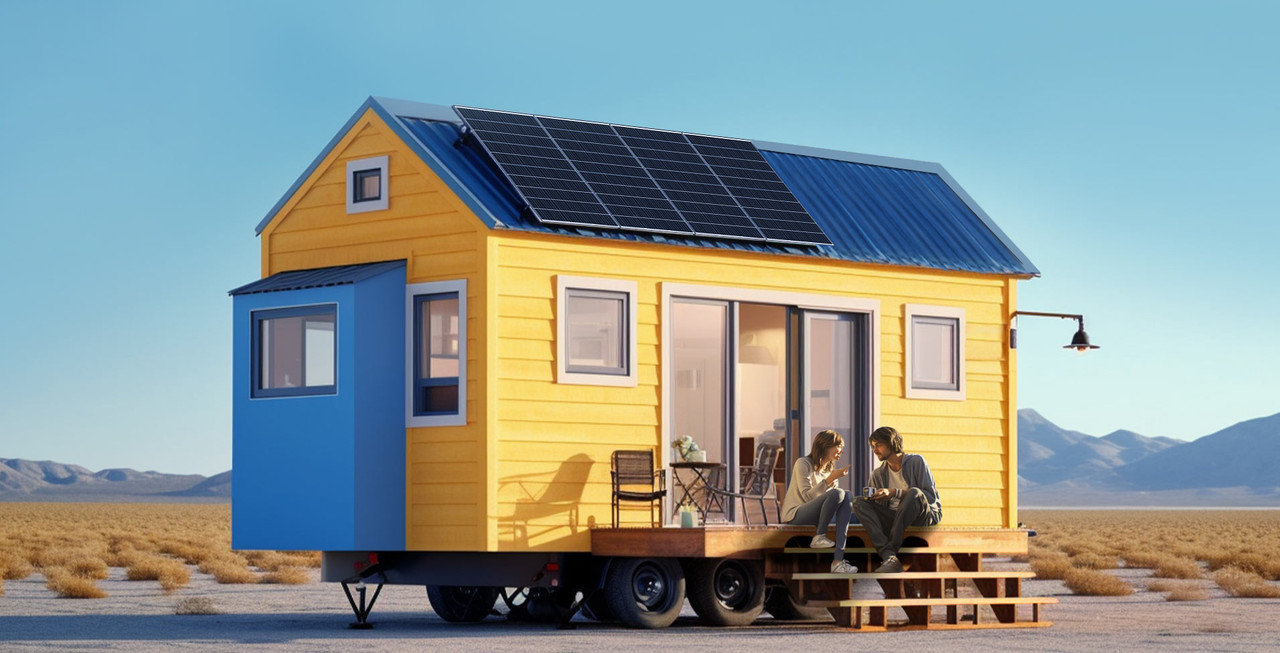The image features a vibrant yellow tiny house on wheels, showcasing various blue accents, including a blue roof and a small blue extension. Prominently, there is a solar panel positioned at the front of the roof. A noticeable metal lamp hangs from the side of the house, illuminating the small wooden porch with three steps leading up to it. On the porch, a man and a woman sit on two small chairs, facing each other across a small metal table. The house has multiple windows and a large glass patio door that offers a glimpse inside. The background reveals a desert-like landscape with scrub brush, mountains, and a clear blue sky, creating a striking contrast to the bright yellow house.